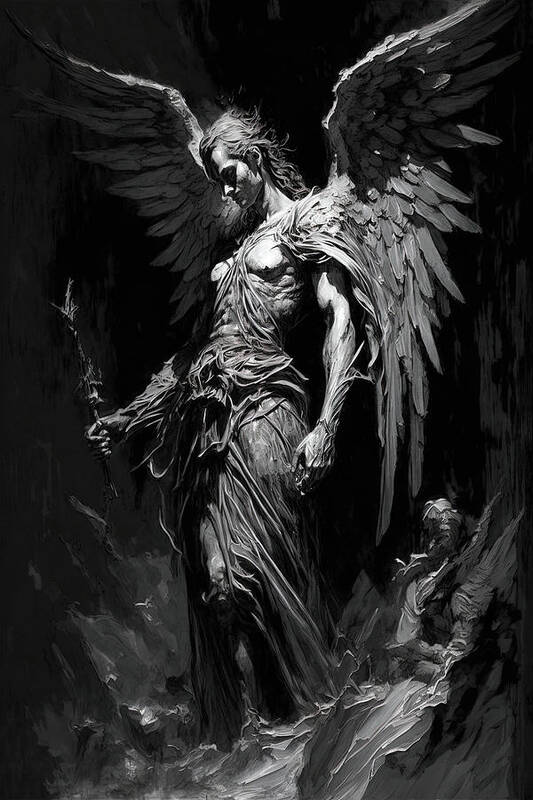This is a highly detailed black and white drawing of an angel, rendered with smooth, precise strokes that could be pencil, charcoal, or digital art. The angel, appearing male based on facial features and musculature, has long, unkempt hair flowing down its back. He is depicted descending a rocky hill, clad in a robe that reveals part of his chest. The robe drapes over his neck, extending below his knees. He holds a handheld staff in his right hand. His left arm hangs by his side. The angel's large wings stretch out majestically, with gradients of gray from dark at the center to lighter at the edges. In the lower left corner of the image, there is another figure, possibly in a military uniform— a cherubic character sitting on a boulder, adding an intriguing element to the composition. The background features dark brush strokes transitioning to lighter grays, creating a dramatic contrast that highlights the angel’s ethereal presence.